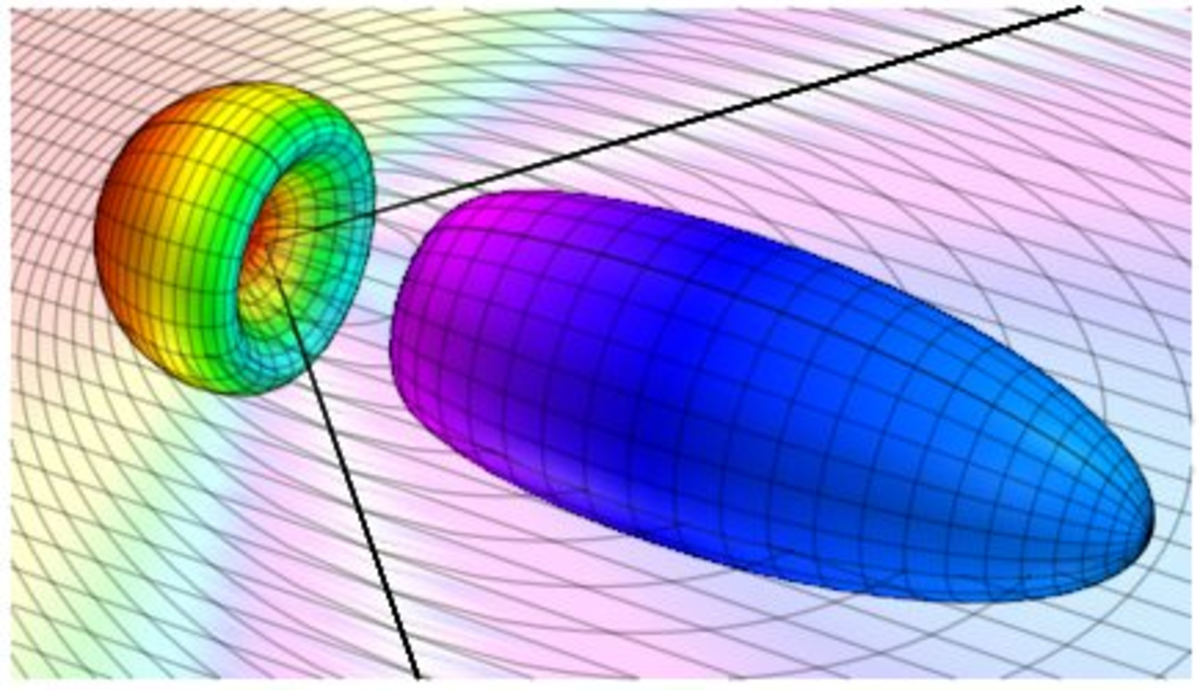This highly detailed, computer-generated image showcases two interlocking, three-dimensional pieces set against a dynamic background of intersecting and swirling lines. The primary piece appears reminiscent of a cup turned sideways, with a rounded, somewhat hollowed-out top. It's vibrantly colored in hues of green, yellow, and orange. Extending from this piece are two black lines forming a V-shape. Nestled within this V is the second object, which closely resembles a blimp or an elongated, oval shape with a digital design. Predominantly blue with purple accents, this object features black linear markings and fits seamlessly into the hollowed space of the first piece. The background enhances the visual complexity with circular and diagonal line patterns, further emphasizing the intricate design and the seemingly stable relationship between the two geometric forms.